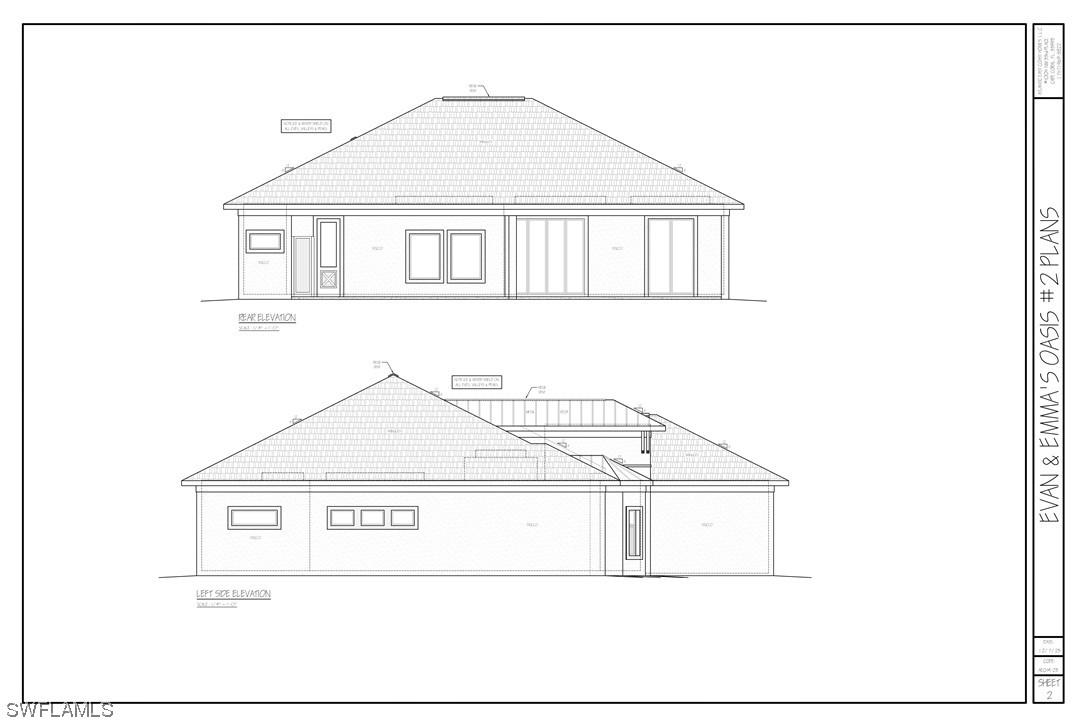The image is a detailed black and white architectural sketch of two sides of a house, depicting both the front and the side views. The front view showcases an arched roof with a flat section on the top. Central to this section are two large windows. Moving left, windows span from the doorway, which resembles a half-screen door with a window on the top half and a screen below, to a solitary window. To the right, a prominent feature includes long vertical windows extending from the roof down to the ground. 

Below, the side view reveals an arched roof peaking in the center on the left. On the wall beneath, a single rectangular window is positioned on the left, while a second rectangular window with three panels is to its right. The bottom left corner of the sketch features the text "S-W-F-L-A-M-L-S" in black, while a vertical sidebar on the right side states “Evan and Emma's Oasis No. 2 Plans.”

The sketches suggest floor plans or blueprints, drawn in pencil, with some additional squares containing information that isn’t clearly legible.